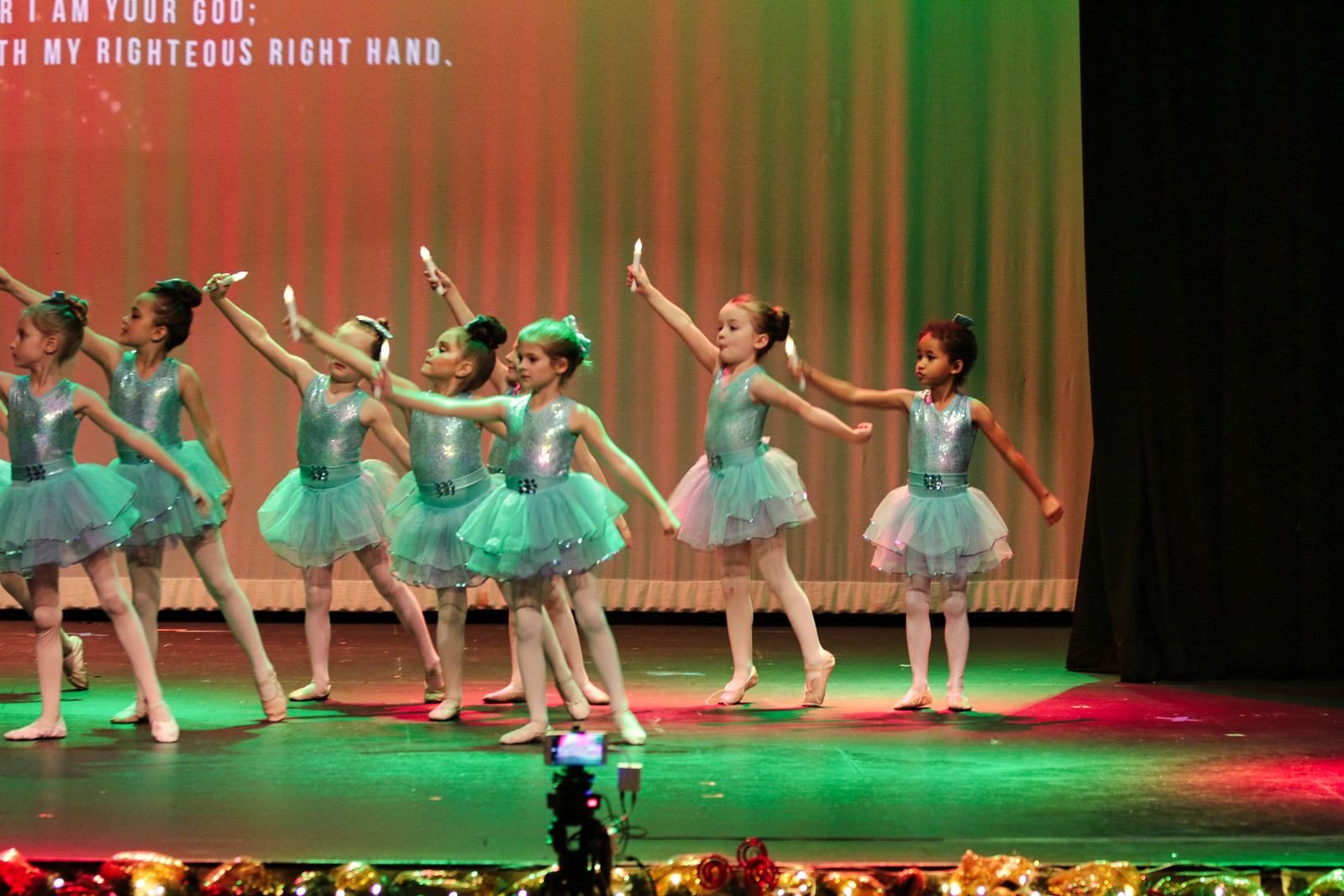In this captivating image of a young ballerina dance troupe during a recital, eight little girls are beautifully posed on an illuminated stage bathed in green and red lights. Each ballerina is adorned in a sparkling mint green bodice with a matching tutu, white tights, and white ballet slippers. Their right arms gracefully extend upwards, each holding an electric candle, casting a gentle glow as they lean to their right. Above them, partially visible text reads, "I am your God with my righteous right hand," against an ombre backdrop of red and green curtains. Alongside the stage, Christmas decorations, such as wreaths adorned with white lights, enhance the festive ambiance. A video camera captures the enchanting performance, adding to the sense of a cherished moment being immortalized.